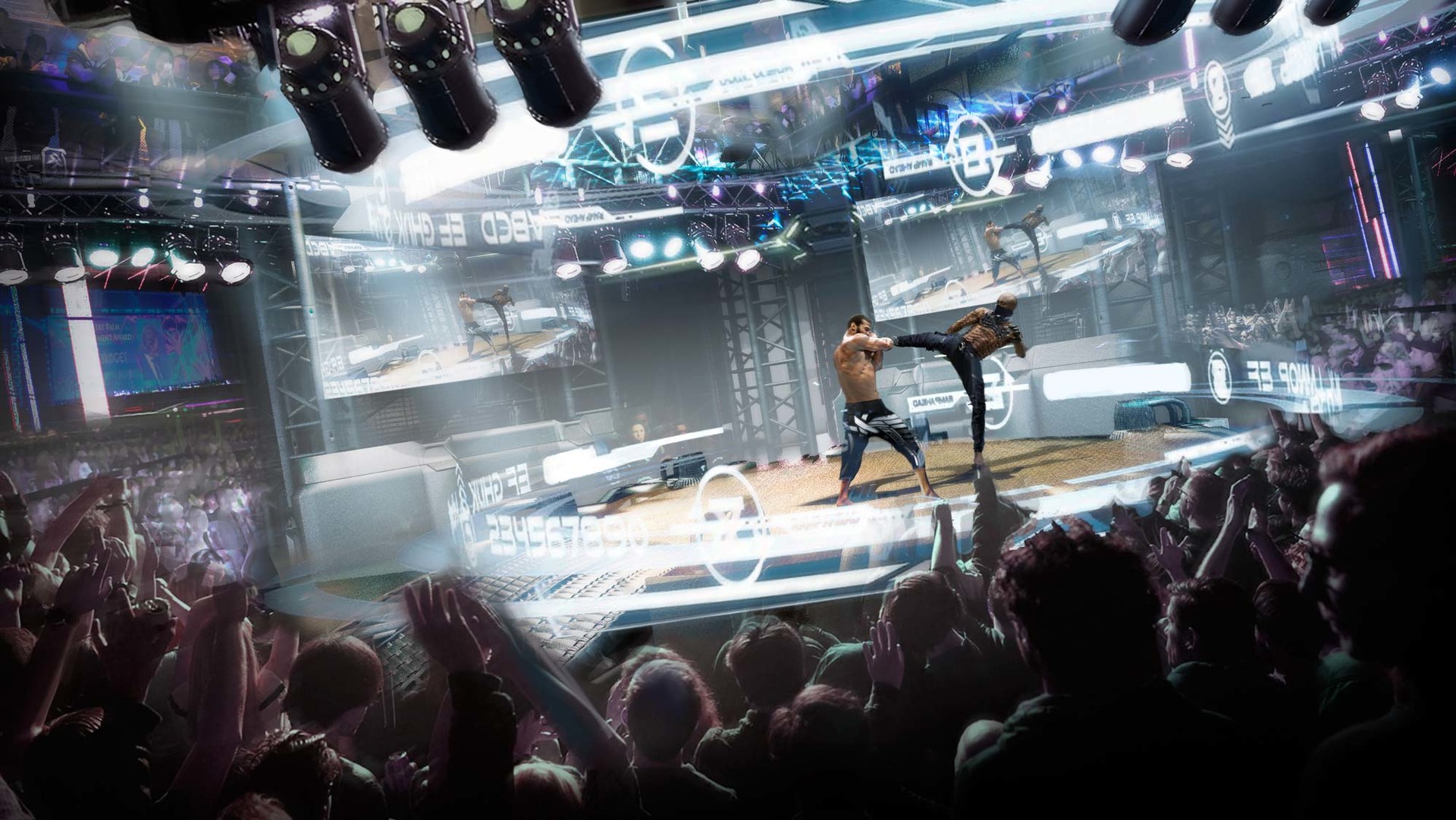The image, possibly an animated or hyper-realistic piece from a movie, cartoon, or video game, showcases an intense, futuristic fight scene. In the center of a brilliantly lit stage flanked by large LCD television screens, two shirtless fighters engage in a dynamic bout. One, an African-American man, delivers a high kick towards the head of his opponent, a Caucasian man, who attempts to block the strike with his arm. Both combatants are barefoot and dressed in dark karate-style pants, with the African-American man wearing black pants and the Caucasian man in white. The stage is encircled by a translucent cage wall, adding to the intense atmosphere. Surrounding the stage is a large, enthusiastic crowd with their hands raised and expressions of excitement, cheering and engaging with one another as they watch the thrilling match unfold.